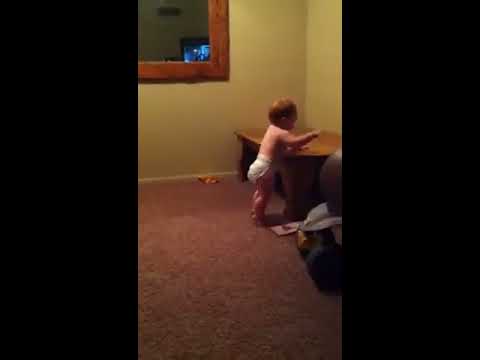In this portrait-oriented photograph, we see a toddler with orangish-reddish hair standing in a living room or children's playroom during the day. The child, wearing only a white disposable diaper, is leaning against a large brown coffee table situated in the corner of a room. The baby is positioned just right of center and faces to the right, leaning slightly against the table. The room features light yellow painted walls and a carpeted floor, which variously appears to be brown or pink. In the upper left corner of the image, a mirror reflects a television or computer monitor with a blue light and black outline. Scattered around the room are several objects, including unidentified items on the floor and a black round object in the foreground. The overall scene captures a quiet, domestic moment in an indoor setting.